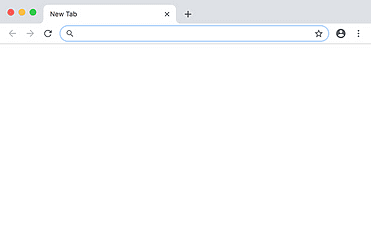This image captures the upper section of a computer screen, showcasing a browser interface. At the very top, a light gray rectangle spans horizontally from left to right. Nested within this rectangle is an active tab, highlighted in white. 

On the left side of this tab, three small circles appear in a row: one red, one yellow, and one green. These circles are typically associated with window controls. Adjacent to these circles, the tab is labeled "New Tab," with the 'N' in "New" and the 'T' in "Tab" capitalized. Towards the center of the tab, there is an 'X' icon, which can be used to close the tab.

Next to this is a '+' icon, which allows for opening additional tabs. 

Moving down to the next section, there are navigation controls: a left-pointing arrow (back), a right-pointing arrow (forward), and a refresh button. Further along, there is a search bar with a star icon at its end, likely for bookmarking. To the right of the search bar are additional icons: a small head-and-shoulders profile indicating a user account and three vertical dots, suggesting a menu or more options.